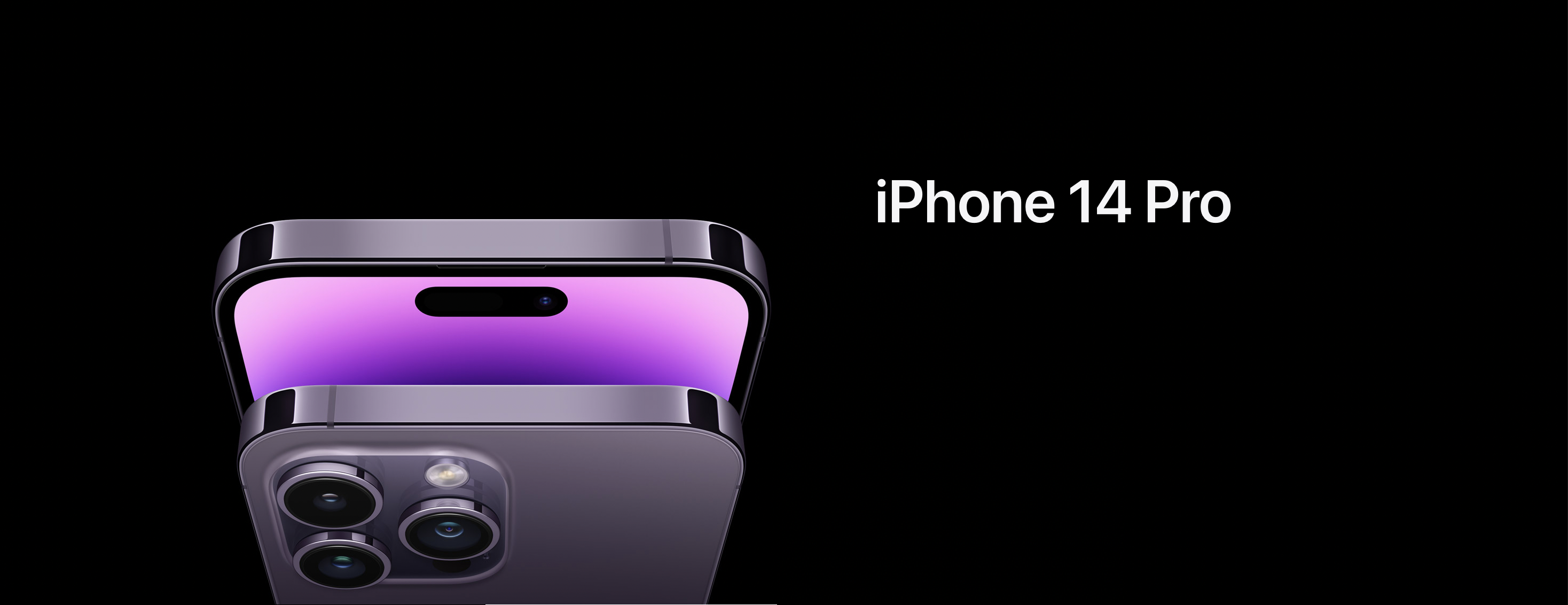Promotional Header Image for iPhone 14 Pro - This promotional image, ideal for a phone store, accessory shop, or even the Apple website, features a sleek, solid black background with a horizontal rectangular orientation. Situated on the right-hand side, about two-thirds of the way up, the text "iPhone 14 Pro" is prominently displayed in white, with a distinctive style: a lowercase "i," followed by uppercase "P," "H," "O," "N," "E," the number "14," and "Pro" with a capital "P". Flanking the text are two images of the iPhone 14 Pro. The front view shows a reflective, glossy black top bezel with a distinct purple screen, though much of this is obscured by the rear view of the phone. The back of the iPhone 14 Pro is showcased in a sophisticated gray color, highlighting its three-camera system and flash sensor.